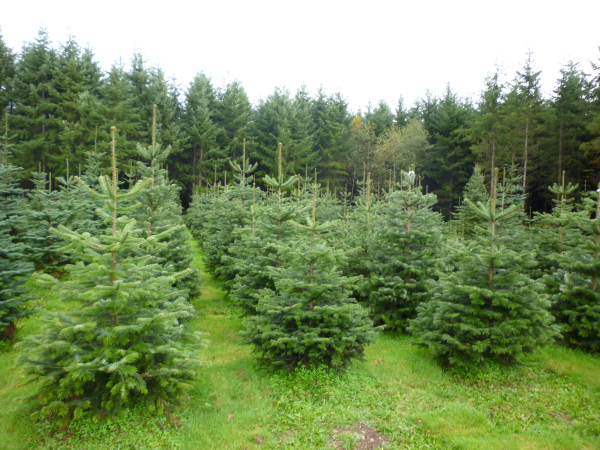The image depicts an orchard of small evergreen trees, meticulously arranged in neat rows spanning several columns from left to right. The trees, characterized by their dark green hue and long, thin needles, feature distinctive brown points at their tops. The foreground reveals a carpet of lush green grass with a few patches of brown dirt, particularly noticeable in the center in front of the first tree. In the background, significantly taller evergreen trees loom, their dark green branches and needles contrasting sharply with the smaller trees in the foreground. The sky above is a luminous white, creating a stark backdrop for the vibrant greens of the orchard. This blend of small and large trees and the orderly rows suggest a managed tree lot, possibly one where Christmas trees are cultivated.